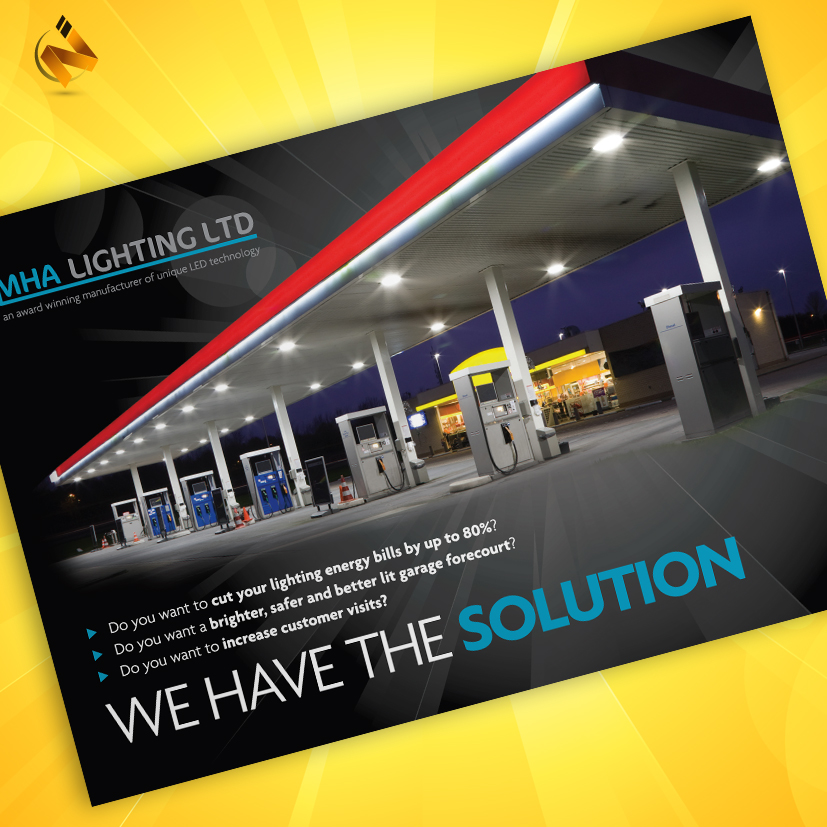The advertisement features a digitally-enhanced, diagonally positioned image of a gas station at night, set against a bright yellow background with rays streaking out like sunlight. The gas station, with its long white canopy and red roof, illuminates the scene through several lights underneath, highlighting multiple empty fuel pumps. The gas station backdrop includes a yellow-lit convenience store. Positioned at the top-left corner is an orange 'N' logo. Above the image, in blue and gray letters, it reads "MHA Lighting LTD: An award-winning manufacturer of unique LED technology." Below that, three bullet points in white lettering ask: "Do you want to cut your lighting energy bills by up to 80%?", "Do you want a brighter, safer, and better-lit garage forecourt?", and "Do you want to have increased customer visits?” The ad culminates in a bold declaration, “WE HAVE THE SOLUTION” with "solution" prominently highlighted in blue letters.